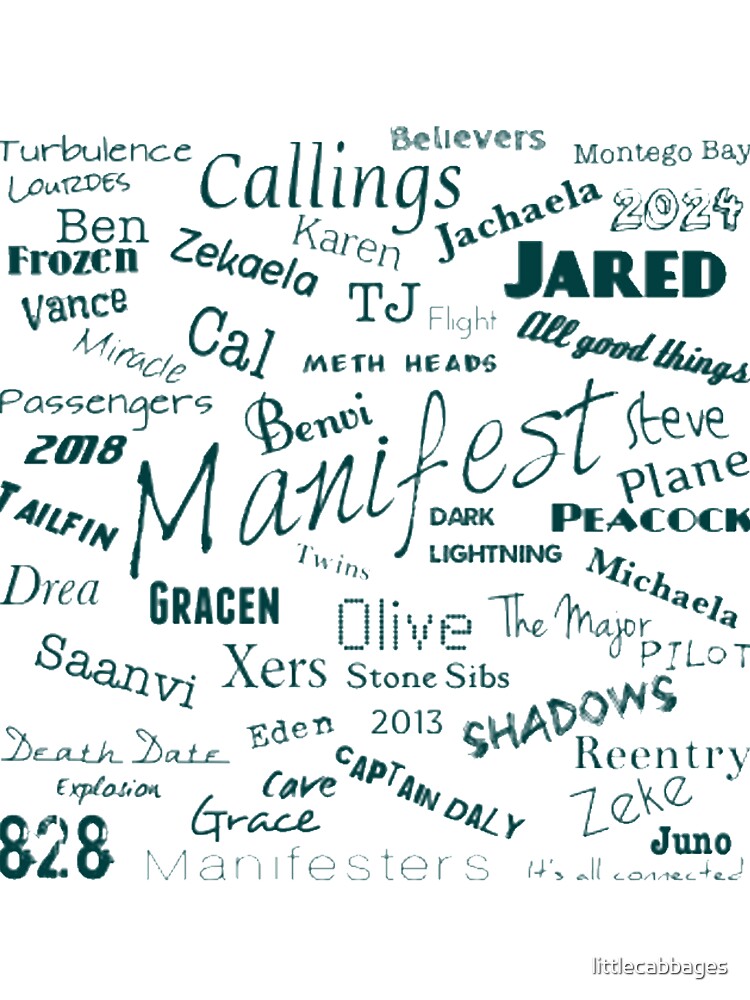The image features an extensive collection of words displayed in various fonts and sizes, all in a dark green color against a white background. Dominating the middle of the picture in a large font is the word "Manifest." Surrounding this central word are numerous others, each in distinct fonts and orientations, including "Turbulence," "Lords," and "Ben" in fancier fonts, "Frozen" in a bold font, "Vance" in a comic font, and "Miracle" in a skinny font. Additional words scattered around include "Passengers," "2018," "Tailfin," "Drea," "Sanvi," "Death Date," "Explosion," "828," "Callings," "Olive," "The Major," "Pilot," "Believers," "Montego Bay," "Jakayla," "2024," "Jared," "TJ," "Meth Heads," "Flight," "All Good Things," "Ben V," "Steve," "Plane," "Peacock," "Dark Lightning," "Michaela," "Twins," "Grayson," "Eden," "2013," "Captain Daily," "Cave," "Grace," "Manifestors," "Shadows," "Reentry," "Zeke," and "Juno." Each word is presented uniquely, contributing to an overall dynamic and varied visual effect. In the bottom right corner is a watermark stating "Little Cabbages."